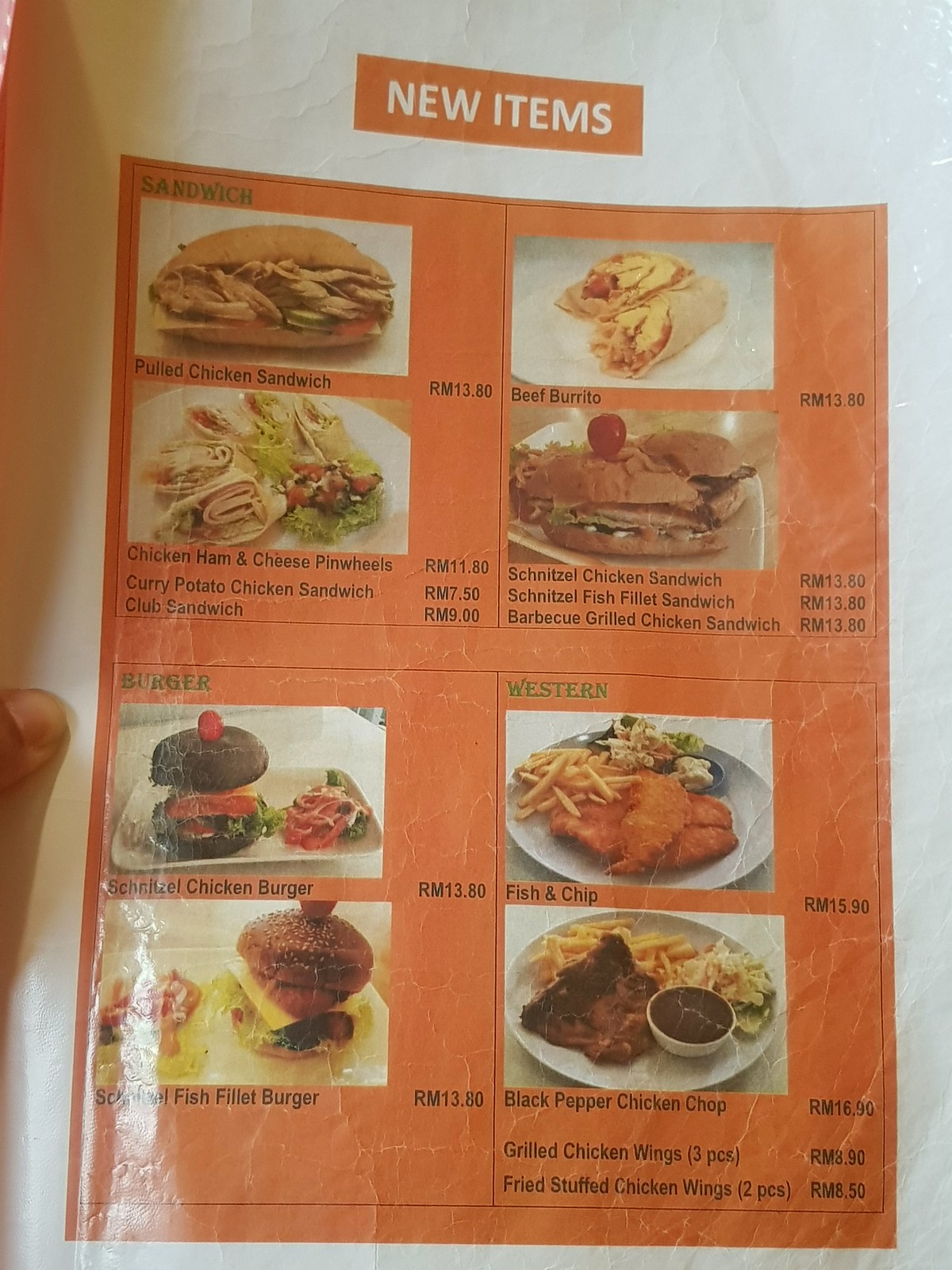The image displays a printed menu on a white background, with a person's finger visible on the left side holding it. The menu has a structured format with items and prices clearly listed. The title "NO ITEMS" is prominently written in all capital letters at the top with an orange background and white type. 

On the left side, there are several food items listed with accompanying pictures:
- "Pulled Chicken Sandwich" 
- "Chicken, Ham, and Cheese Pinwheels" 
- "Curry Potato Chicken Sandwich"
- "Club Sandwich"

The prices on the left side range from $9.00 to $13.80.

To the right, the menu lists:
- "Beef Burrito" 
- "Schnitzel Chicken Sandwich" 
- "Schnitzel Fish Fillet Sandwich" 
- "Barbecue, Grilled Chicken Sandwich"

The items on the right are mostly priced at $13.80.

Below the pictures on the left, it continues with:
- "Burger" 
- A "Schnitzel Chicken Burger" shown on a white dish, priced at $13.80
- A "Schnitzel Fish Fillet Burger," priced at $13.80

To the right under the section marked "Western," it features:
- "Fish and Chips" for $15.90
- "Black Pepper Chicken Chop" for $16.90

Below these items, it's noted:
- "Grilled Chicken Wings, three pieces" for $8.90
- "Fried Stuffed Chicken Wings, two pieces" for $8.50

Each section is thoughtfully organized with clear images and consistent pricing, ensuring an easy and pleasant browsing experience for potential customers.